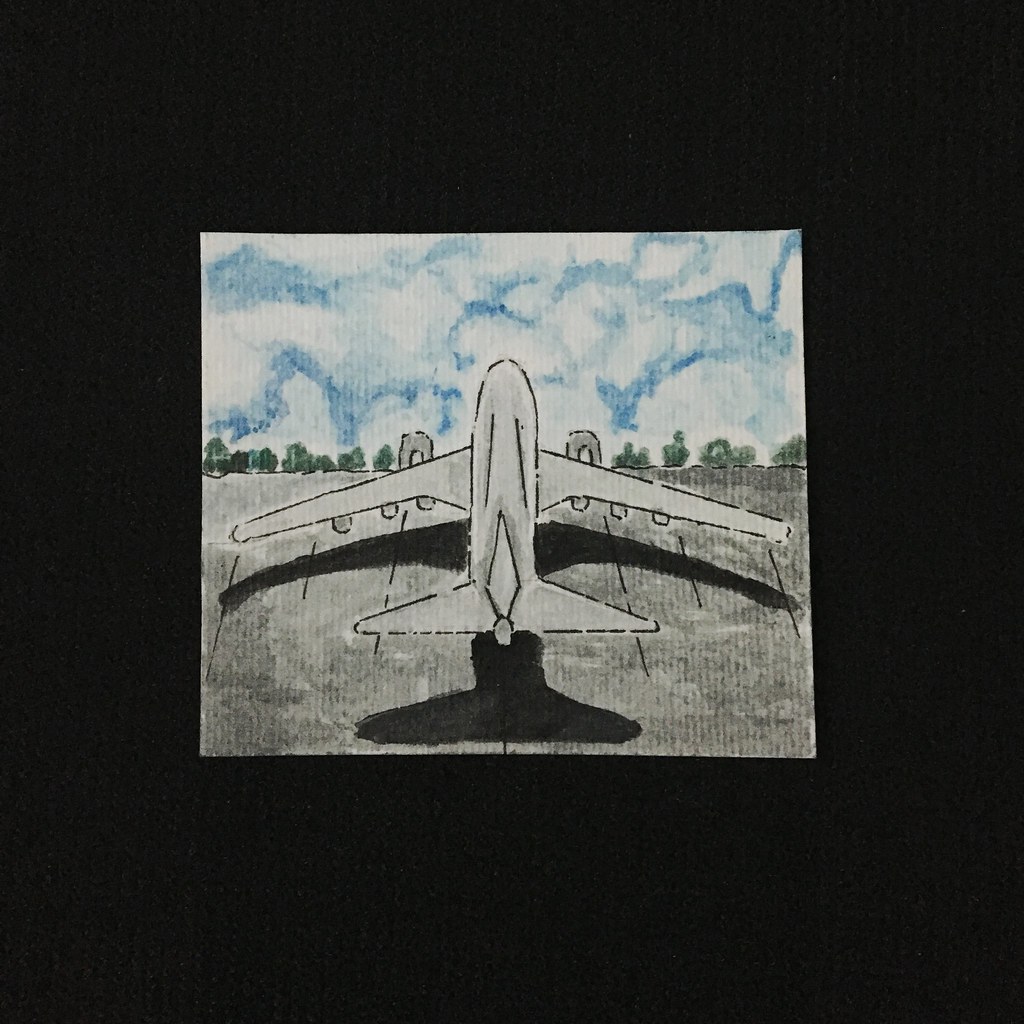A sleek, gray airplane appears in the center of the image, flying forward against a vivid blue sky dotted with white clouds. The ground beneath the plane is shrouded in darkness, adding a striking contrast to the vibrant sky. Surrounding the plane, the sky displays a gradient from deep blue to lighter hues. In the middle distance, a cluster of green trees adds a touch of nature to the scene. The airplane, featuring prominent jet engines and sturdy wings, has multiple lines attaching it to the ground, possibly indicating it is part of an aviation display or test scenario. A flag can be seen near the plane, adding to the overall sense of precision and pride in this detailed aviation shot.